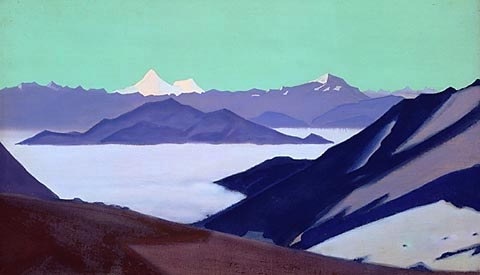This painting, titled "Fog in the Mountains," was created by Nicholas Roerich in 1945. It showcases a stunning mountain landscape using simplistic shapes and flat colors. The foreground features a prominent brown rock formation on the bottom left, contrasted by a navy blue rock formation with gray streaks on the right. Positioned behind these elements is a striking blue mountain range, slightly left of center.

Further into the distance, a horizon of purple mountain ranges emerges, accompanied by a few birds flying overhead, adding a touch of life to the serene scene. The distant mountains are crowned with a snow-covered peak and a slightly shorter, adjacent peak. The entire background is enveloped in an aqua green sky, imparting an ethereal quality to the painting.

The mountains display varying hues of purple, reflecting the changing light as the sun interacts with the terrain. This artistic presentation leans towards Russian realism, emphasizing the grandeur and mystique of the natural world rather than striving for a purely realistic depiction. The white snow on the mountains, especially prominent in the further ranges, adds to the ethereal beauty of the scene, making it appear that the viewer is peering through layers of fog and time.